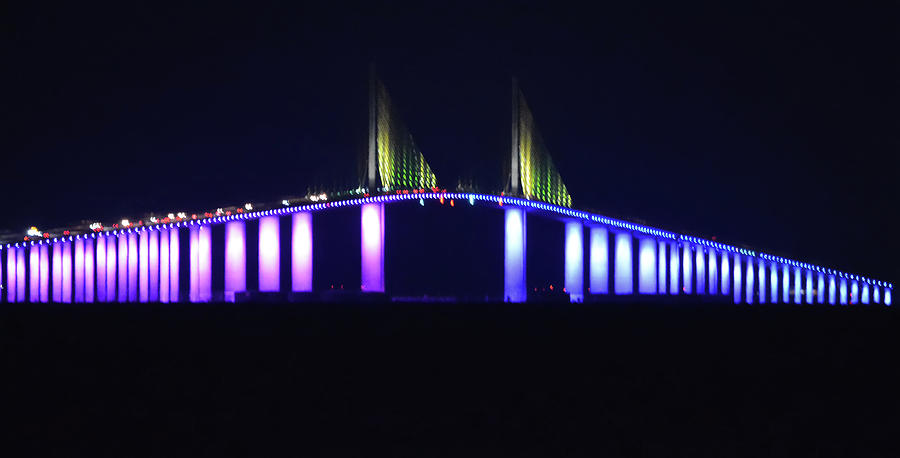This nighttime photograph captures a large, horizontal bridge adorned with vibrant LEDs, standing out against a pitch-black sky and foreground. On the left side of the bridge, neon purple lights glow vividly along the structure and reflect off the sturdy pillars beneath, which likely descend into unseen water. The right side of the bridge contrasts with a striking blue illumination that extends across the pylons and side of the bridge. Atop the bridge, green and occasional yellow neon lights shimmer, creating a vivid spectacle. Numerous cars, primarily on the left side due to the angle, travel along the bridge, their sides faintly visible. The detailed lighting—from purple and blue to green and yellow—enhances the bridge's grand structure, making it a central and captivating element in the dark, serene scene.